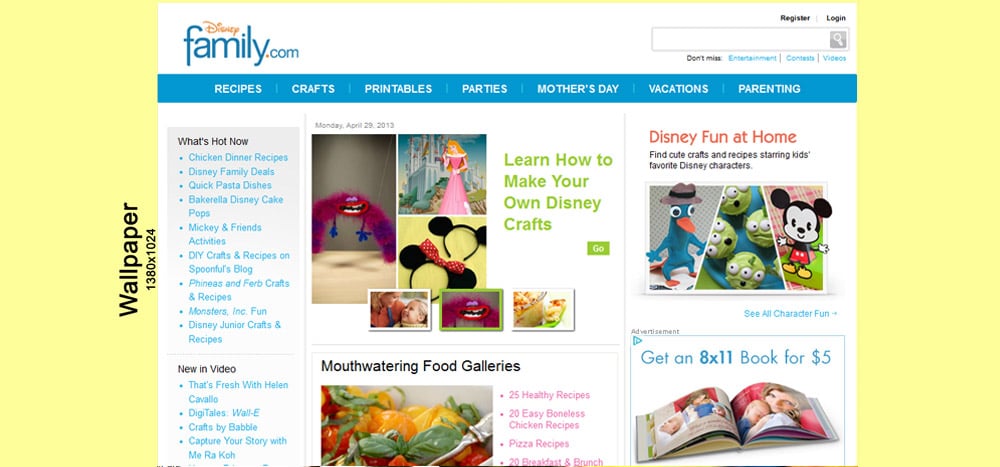The image displays a vibrant webpage layout with various sections and colorful elements. On the left and right sides of the page, there are light yellow boxes. The yellow box on the left features the text "Wallpaper 1380 x 1024". In the center, a large white box prominently shows the logo "DisneyFamily.com" along with options to "Register" and "Login", and a search box for users to navigate the site. Below this, there are several navigation options listed in a small blue box, including "Recipes", "Crafts", "Printables", "Parties", "Mother's Day", "Vacations", and "Parenting".

Adjacent to this, another light blue box labeled "What's Hot Now" lists trending items. A separate section marked by a small dividing line highlights "New" and "Video", showcasing the latest video uploads. 

To the right, the page is dated "Monday, April 20, 2013" with several pictures displayed: one shows a quirky little monster character with a red body and blue legs shaped like stars, another a small square image of a Disney princess in pink, and a tiny square of Mickey and Minnie ears. Below these, three smaller images are arranged in a row.

Further down, a box showcases a visually appealing gallery of "Mouth-Watering Food", featuring an enticing image of a delicious dish and promoting recipes with the caption "Learn how to make your own Disney crafts" in green text. A small green button labeled "Go" is also present for quick access.

On the right side, a pink section titled "Disney Fun at Home" invites visitors to find cute crafts and recipes starring favorite Disney characters, accompanied by three small images of Disney-themed cakes and cookies. Finally, the last box on the page has an upper left corner triangle announcing "Get an 8 by 11 book for $5" and features an illustration of an open book.